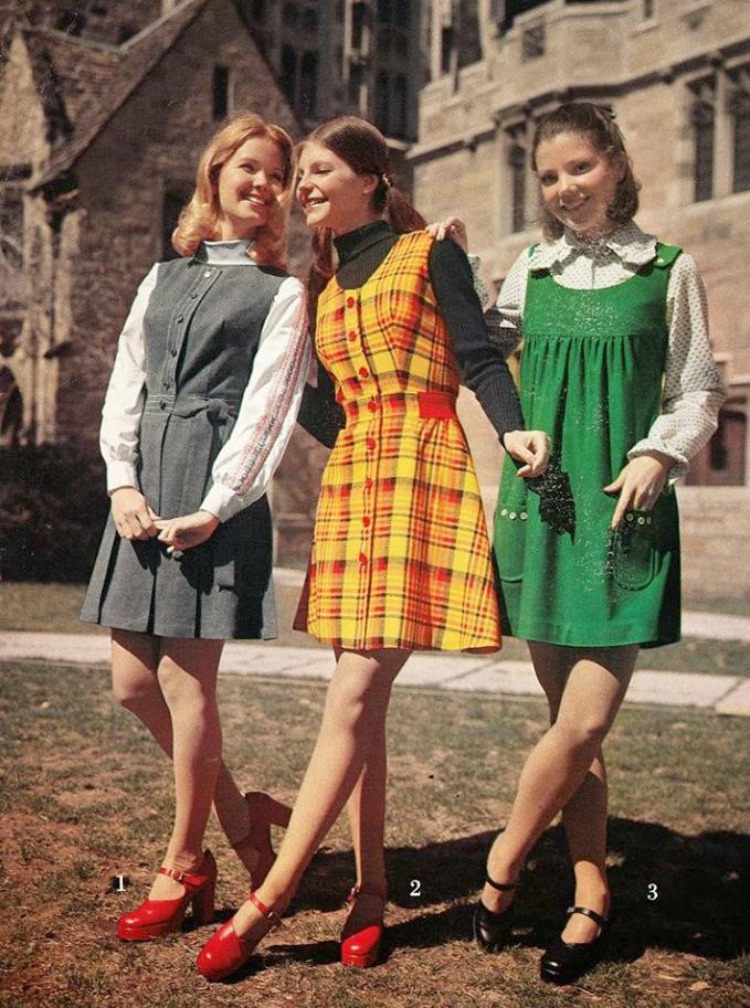This photograph features three young women, likely in their late teens or early twenties, standing on a grassy area in front of a stone or sandstone-colored brick building with numerous arched windows, suggesting it could be a university or a Tudor-style mansion. The building appears to have at least two to three levels. The women are posed in a row with numbers 1, 2, and 3 denoted beneath their feet, from left to right.

The woman on the left, labeled as number 1, has blonde hair and is wearing a gray jumper-style dress that is buttoned down the front over a lightly plaid white and tan shirt. Her dress is pleated and ends just above the knee. She has on red-heeled, platform Mary Jane-style shoes. The middle woman, number 2, has straight brown hair pulled back in ponytails and is dressed in a mustard yellow and brown plaid dress with red buttons, over a dark brown turtleneck sweater. She is also wearing red platform shoes similar to the first woman. The woman on the right, labeled as number 3, has neck-length brown hair and is wearing a green pinafore-style dress with a wide yoke over a long-sleeve white blouse with a Peter Pan collar. Her left leg is crossed over her right shin, and she is wearing black platform Mary Jane-style shoes.

All three women are smiling, with the woman on the right looking directly at the camera while the other two glance sideways with cheerful expressions. The overall image evokes a sense of youthful joy and camaraderie, characteristic of young women modeling collegiate wear from the late 1950s or early 1960s.